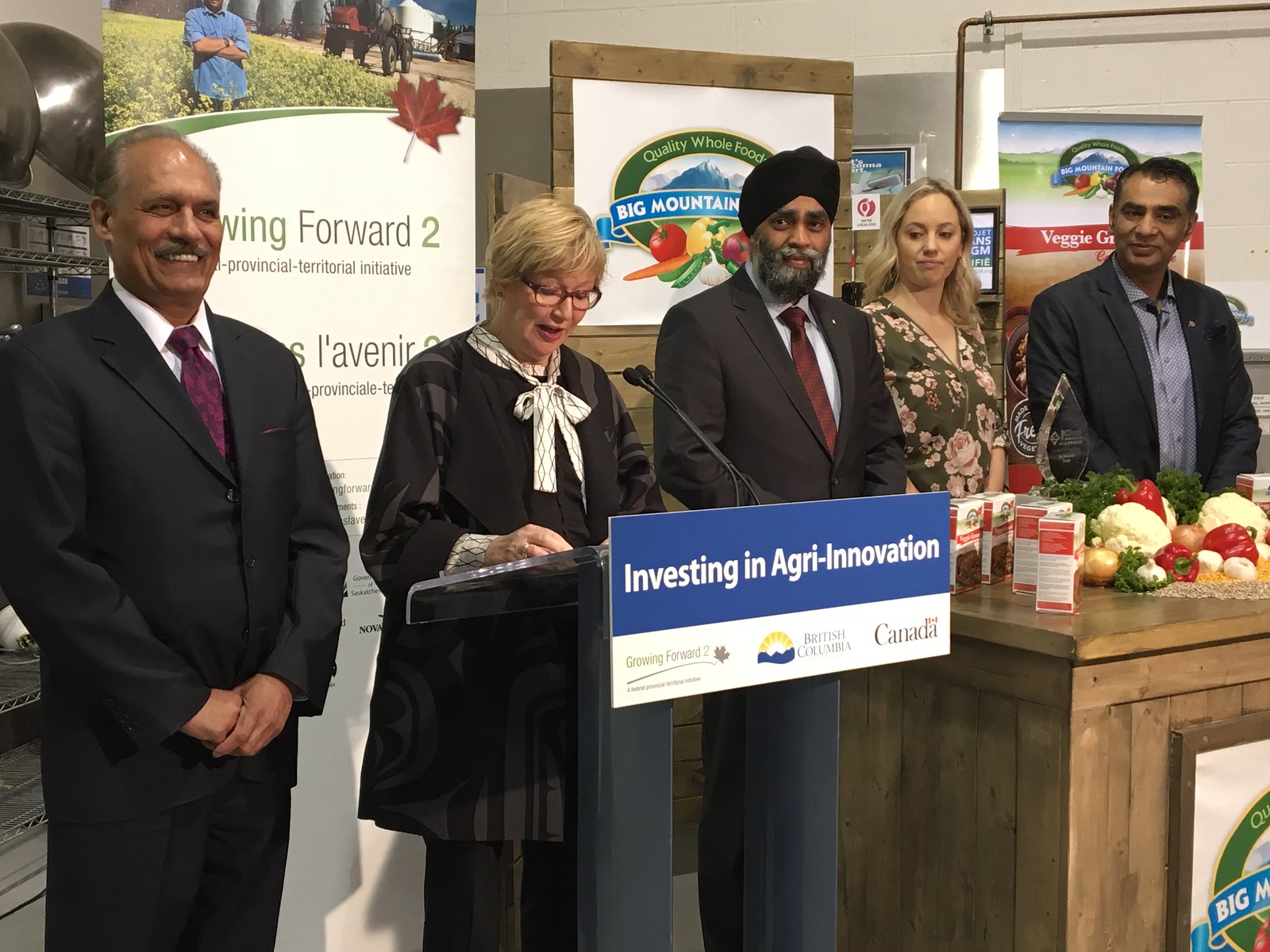In the image, five individuals are standing on a stage, giving a presentation. In the center, a woman with blonde hair and glasses is speaking at a podium that reads "Investing in Agri-Innovation" with "Canada" below in white font on a blue background. She is wearing a black suit jacket, black pants, and a shirt adorned with a bow at the front. Flanked to her right is a man wearing a turban, a gray suit, a blue shirt, and a red tie, and another woman with long blonde hair, wearing a green dress with pink flowers. On her left stands a man with gray hair, a blue suit, white shirt, and purple tie, smiling with his hands folded, whereas the man furthest to the right, in a gray suit jacket and a blue button-down shirt, appears more serious. Behind them, signs in both English and French mention "Quality Whole Foods" and "Big Mountain," featuring images of mountains and various vegetables. A table laden with an assortment of fresh, cut-up vegetables is also visible near the woman in the flower dress, emphasizing an agricultural theme.